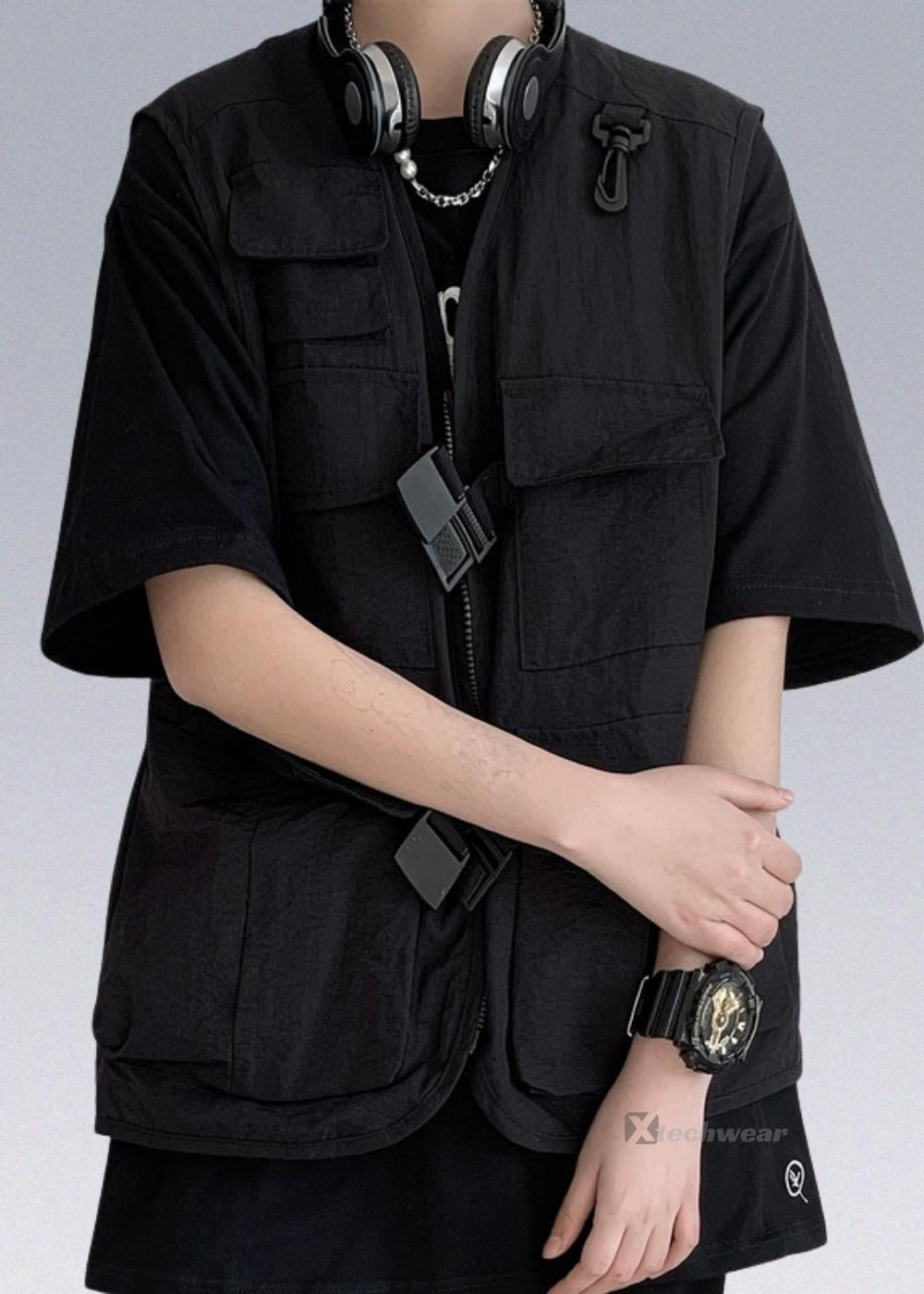The detail-rich photograph captures the upper body of a younger individual, presumably Caucasian, dressed in techwear street fashion. The image centers on a person with very light, pale skin, wearing a medium short sleeve black t-shirt underneath a distinctive black vest adorned with numerous buckles, pockets, and straps, reminiscent of military uniforms. The heavy, elaborate overall attire is complemented by a few key accessories: a pair of black headphones around the neck, a substantial, mechanical black wristwatch on the left wrist, and a silver chain necklace. The individual appears to be slightly slouched, contributing to a casual, disengaged posture. The background is a solid gray, which helps to highlight the dark tones and detailed textures of the techwear ensemble.